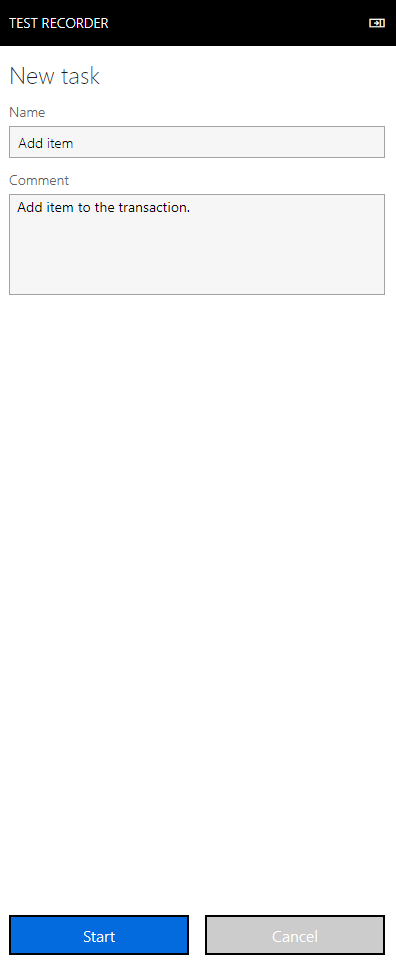In the screenshot, the interface of a test recording application is prominently displayed. At the top, occupying the title bar, is the label "TEST RECORDER" in all capital letters, with white text set against a black background, creating a stark contrast. Directly below this title bar is a section labeled "New Task" with a capital 'N'.

Further down, you find a text field for naming the task, followed by an input bar labeled "Add Item" with a capital 'A'. Below this is a section titled "Comment," and an adjacent rectangular input box prompting the user to "Add Item to the transaction."

At the bottom of the interface are two buttons for user interaction. The "Start" button is in a blue rectangular box with white text, while the "Cancel" button is in a gray rectangular box, also with white text. On the right-hand side of the title bar, next to "TEST RECORDER," is an icon resembling a forward button. The entire interface is set against a clean, white background, enhancing readability and user interface clarity.